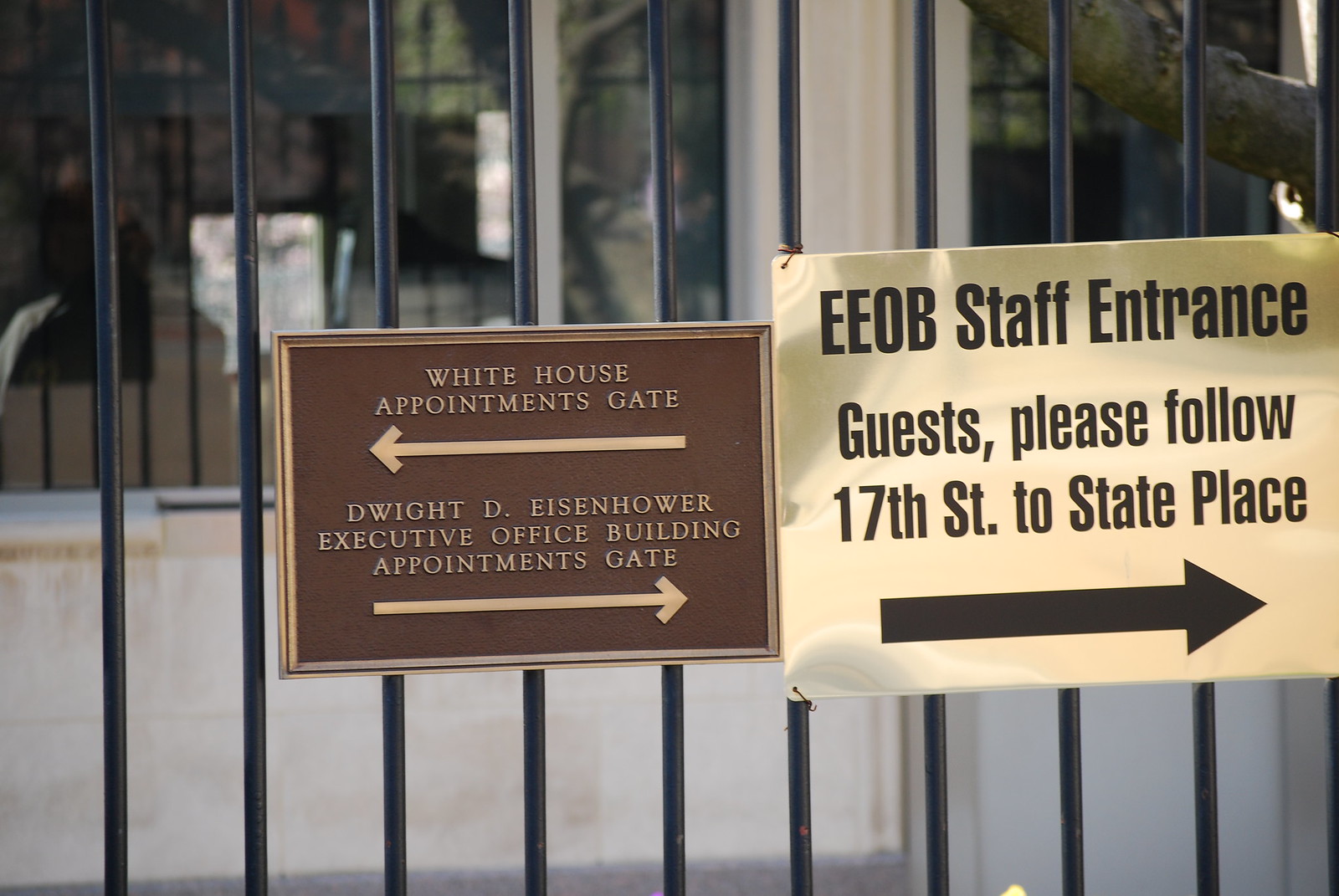The close-up photograph depicts a wrought iron fence with prominent black vertical bars. Attached to the fence are two distinct signs, one on the left and one on the right. The left sign is rectangular with a brown background and a border that appears to be gold or bronze. It reads "White House Appointment Gate" with a white arrow pointing left, followed by "Dwight D. Eisenhower Executive Office Building Appointment Gate" with a white arrow pointing right. The text and arrows on this sign are in a gold or bronze font. The right sign is a rectangular white sign encased in a plastic cover, bearing black text that reads, "EEOB Staff Entrance. Guests, please follow 17th Street to State Place," accompanied by a black arrow pointing to the right. The background reveals a white plaster or concrete building with a couple of windows reflecting trees and a cream-colored brick wall beneath. Additionally, a tree limb is visible in the top right corner of the image.